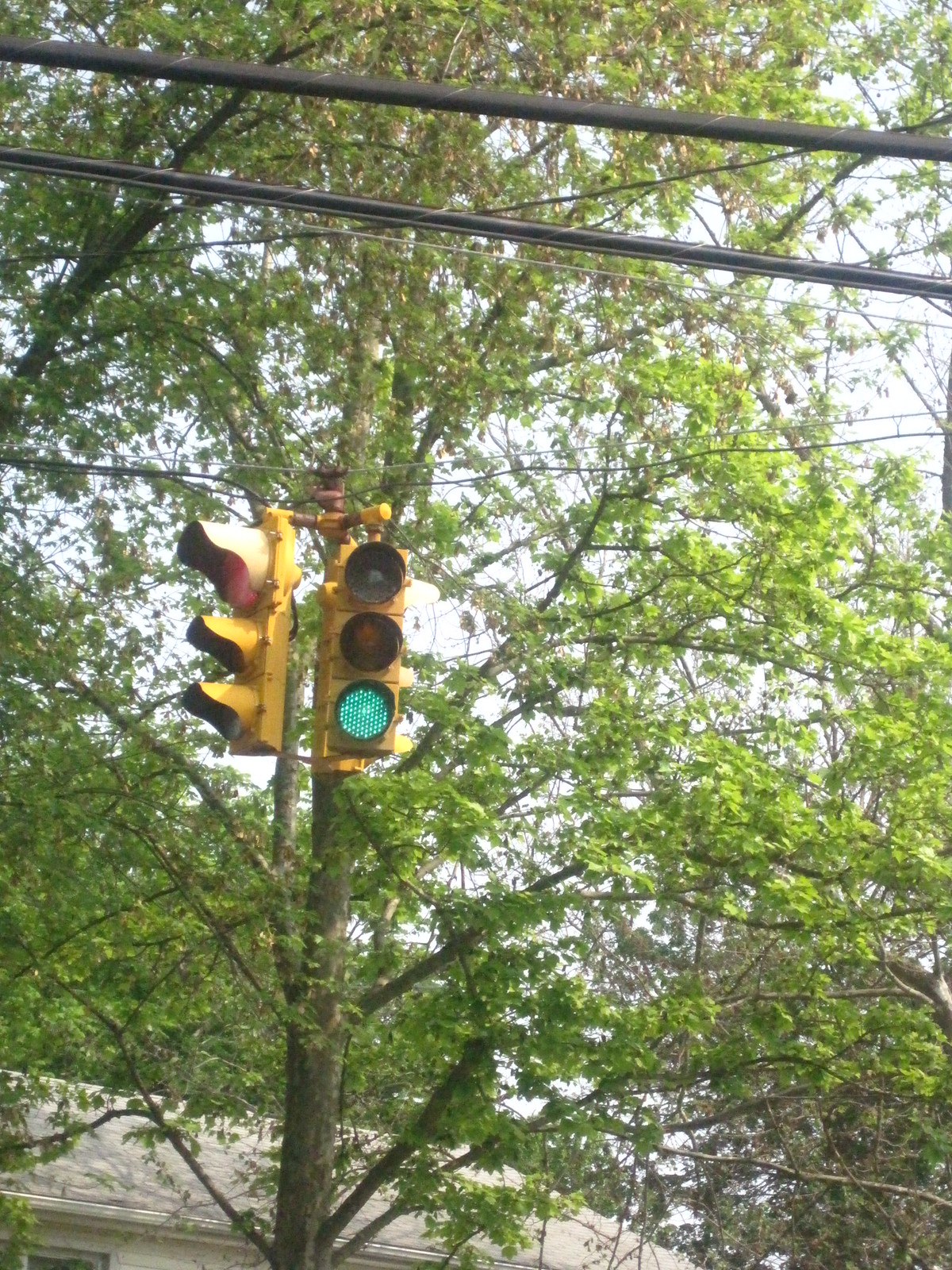In the foreground of the image, a yellow stoplight is prominently displayed, with the green light illuminated for forward traffic and the red light illuminated for side-to-side traffic. The background features a lush tree with vibrant green leaves and sturdy brown branches, partially obscuring a house behind it. Overhead, several wires stretch across the top of the photograph, adding an urban element to the scene.